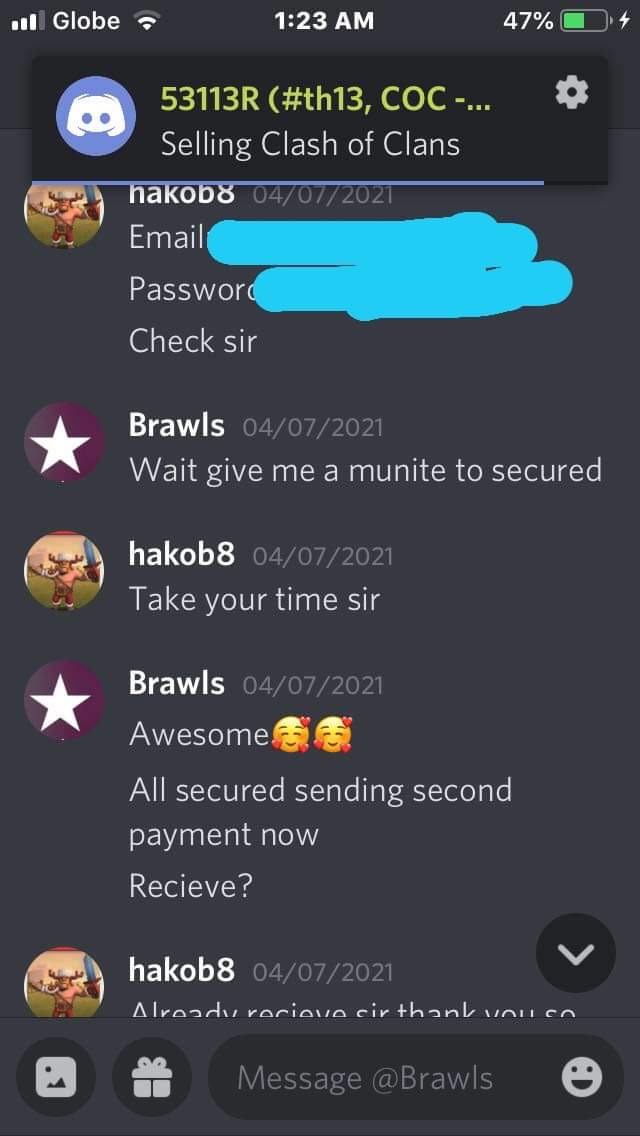This image depicts a vertically oriented screenshot of a smartphone with a black background. At the top of the screen, the status bar shows it's 1:23 AM with a battery level of 47%, and the device is connected to a service called "Globe." The primary focus of the screen is a conversation within a messaging app about selling a Clash of Clans account, indicated by an icon and text that reads "Selling Clash of Clans". 

The messaging thread features an exchange between two users: HackoB8 and Brawls. HackoB8, represented by an icon, sends a message that states, "Email Password Check Sir," with the actual email and password neatly redacted in blue for privacy. Brawls, symbolized by a purple circle with a star, replies shortly after with, "Wait, give me a minute to secured." HackoB8 then reassures with, "Take Your Time Sir." Following that, Brawls responds with enthusiasm, "Awesome, all secured, sending second payment now," accompanied by two heart face emojis. HackoB8 promptly confirms, "Already received Sir, Thank you."

Below this detailed exchange, the screen includes a text input field indicating readiness for the next message.